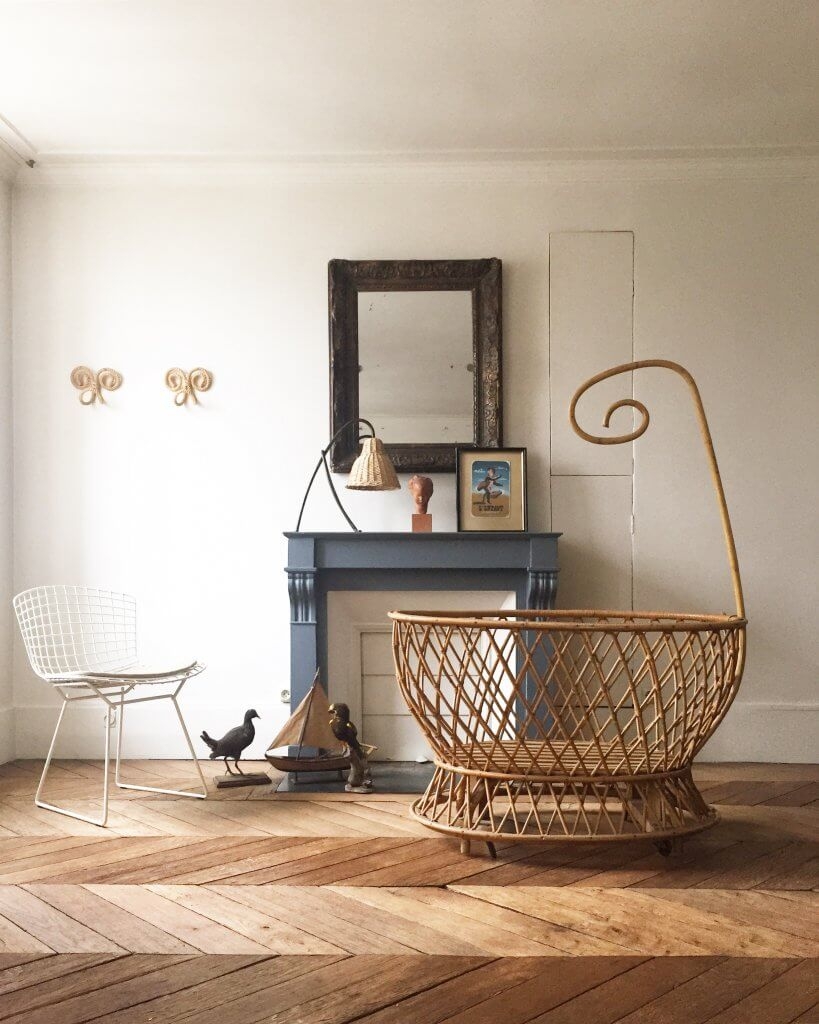This vertically aligned rectangular image depicts a tastefully decorated living room with white walls and ceiling, creating a bright and airy atmosphere. The floor is laid with a zigzag-patterned, alternating dark and light wood tiles, forming distinct V shapes. Central to the wall is an antique-style mirror featuring a brown and gold frame. Beneath the mirror is a slate-colored fireplace mantle, devoid of fire, backed by a walled-off white interior. Atop the mantle, a small lamp with a white bell-shaped shade, a brownish bust, and a framed picture – although indistinct in detail – create a charming arrangement. The hearth in front of the fireplace holds a model ship with two white sails flanked by two bird sculptures, one resembling a peahen and the other possibly a songbird or parrot. On the left side, a white metal chair with a modern, mesh-like back stands on the floor. Opposite, on the right, there is an unusual large wicker chair, almost resembling a bassinet, complete with a tall, curling arm, but lacking a cushion. Additionally, two decorative, bow-like hooks adorn the left wall, adding to the room's quirky elegance.